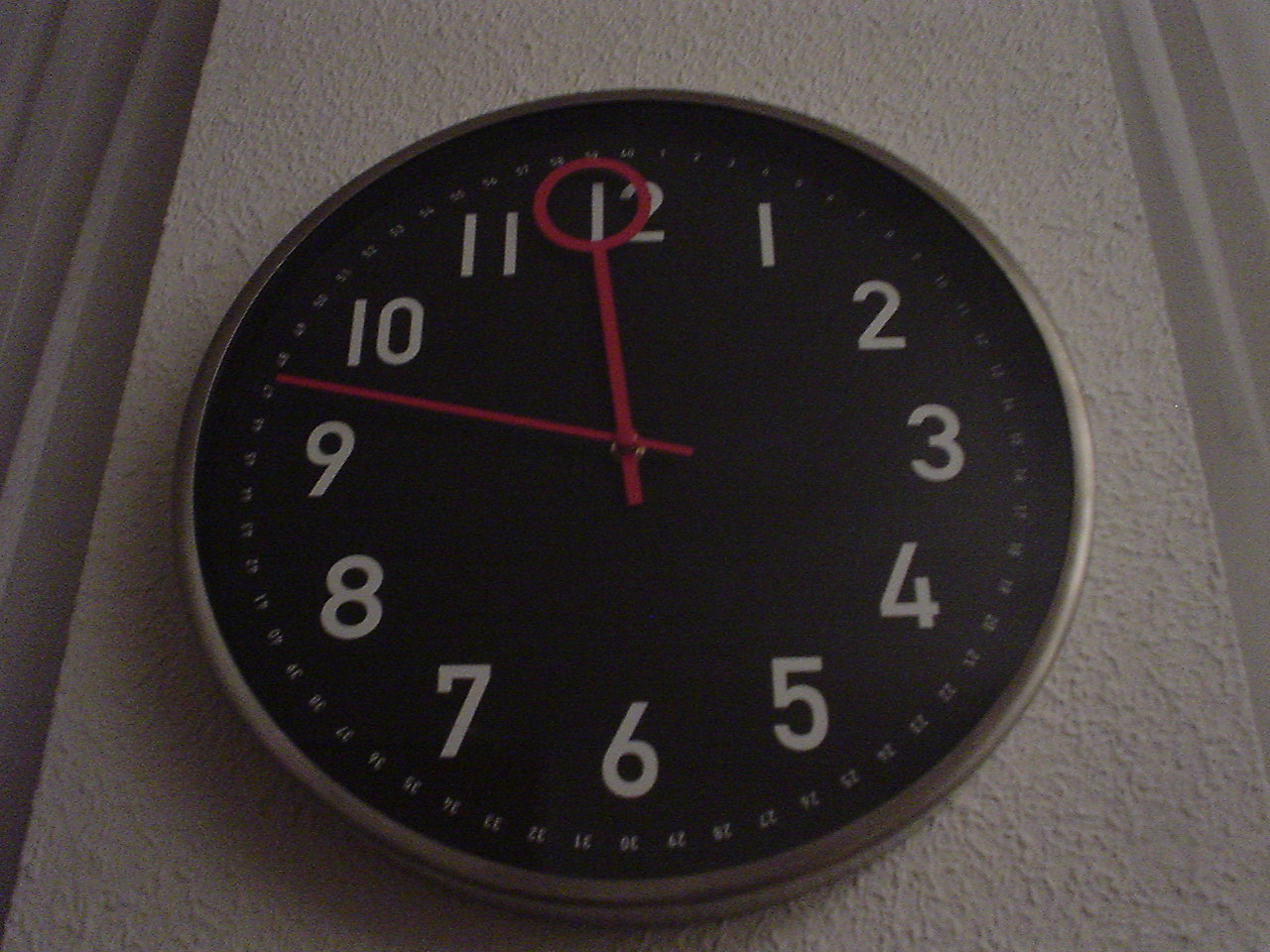This image features a clock mounted on a gray, spackled wall, giving the surface a textured, non-smooth appearance. The clock has a sleek silver rim and a white clock face. Prominently displayed are large numbers marking the hours, with tiny increment numbers between them, likely counting up to 60 for seconds or minutes. The clock's hands are notably unique, with the minute hand resembling a bubble wand, featuring a large circular loop at its tip, adding an unconventional and distinctive touch to the timepiece's design.